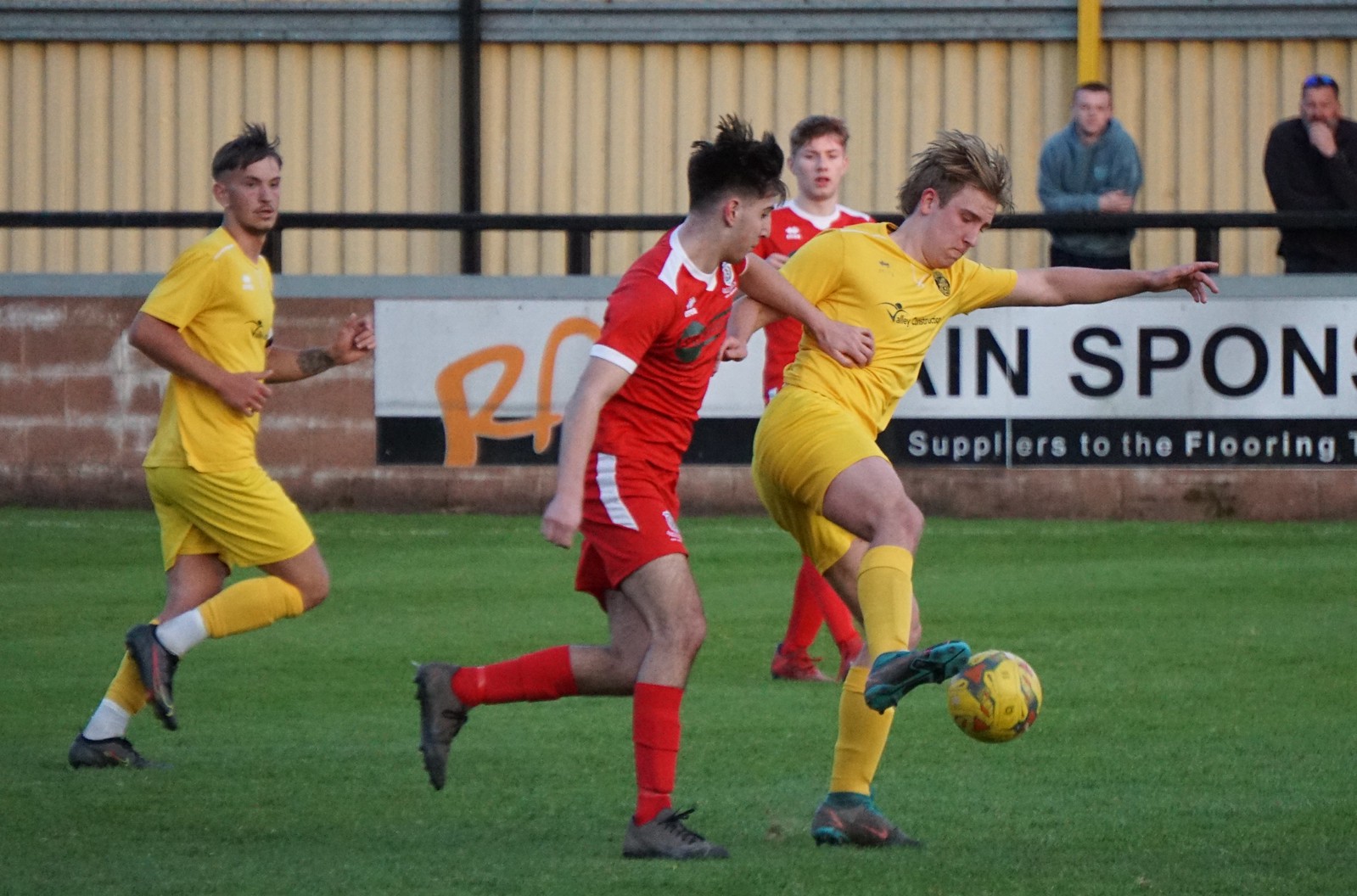The photograph captures an intense soccer match played on a field with vibrant green turf. Four players are on the field: two in bright yellow jerseys, shorts, and long socks, and two in red jerseys with white accents and matching red shorts and socks. In the image, a player in yellow is actively kicking a multi-colored soccer ball—yellow, black, and red—while a red-clad player challenges him from his left side. Another red player is positioned slightly behind, and a second yellow player is situated to the left side of the field.

In the background, a brick wall serves as a boundary, adorned with a banner featuring black letters. Above the wall, two spectators stand against a black railing, one wearing a blue jacket and the other in a black jacket, both intently watching the game. Behind the spectators, a cream-colored wall with gray lines and a gray border can be seen, adding depth to the scene. The natural daylight provides a sharp, clear image of this dynamic moment in the soccer match.